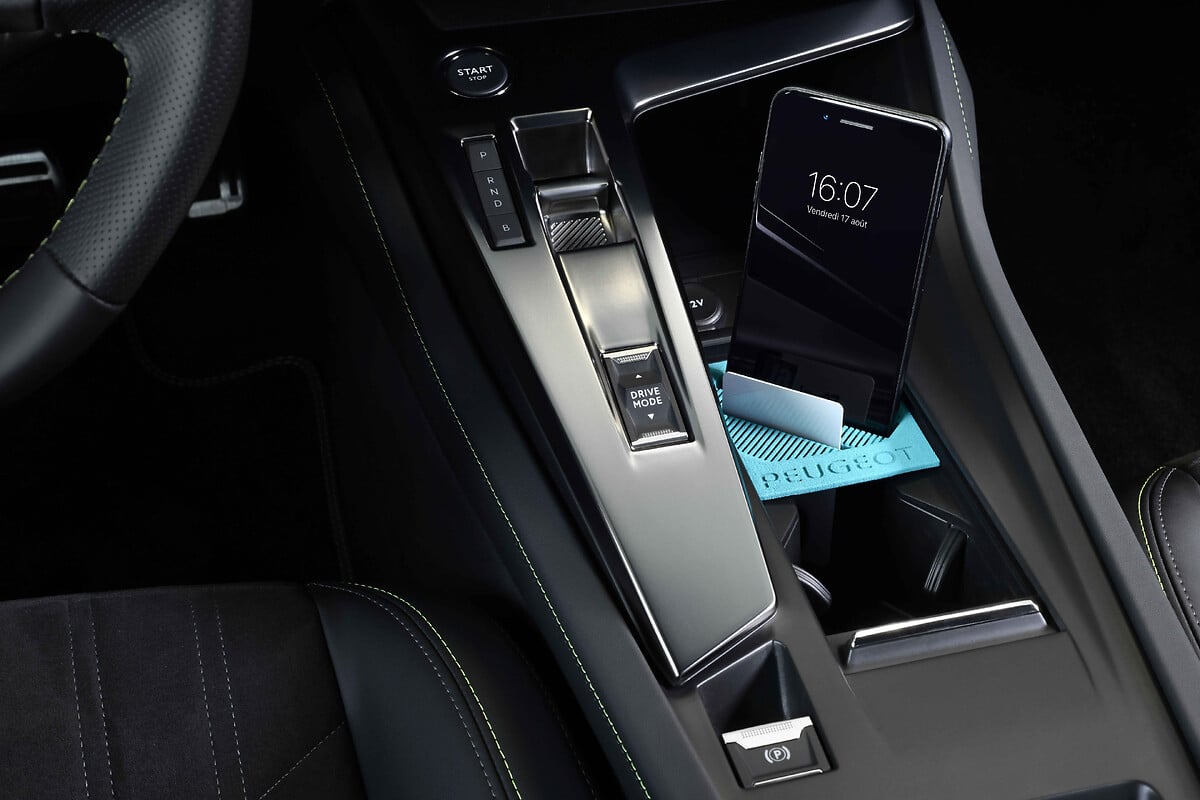This detailed photographic image captures the interior of a car, focusing primarily on the front section. The background features black leather seats on both the left and right-hand sides. The top left corner reveals the edge of a black steering wheel and the driver's seat. Centered in the image is the console area, dominated by a stick shift labeled "PRNDR" for park, reverse, neutral, drive, and another mode. Adjacent to the stick shift is a knob labeled "P" and another one marked "2V."

A smartphone, black in color and mounted on a turquoise blue stand, displays the time "16:07" and the text "Vendredi 17," indicating Friday the 17th. Beneath the smartphone, a piece of paper with the word "Peugeot" in blue and black is visible. The car's interior features various buttons, including one for "Drive Mode" and a start/stop button, all set against sleek, modern design elements in a predominantly black and grey color scheme.